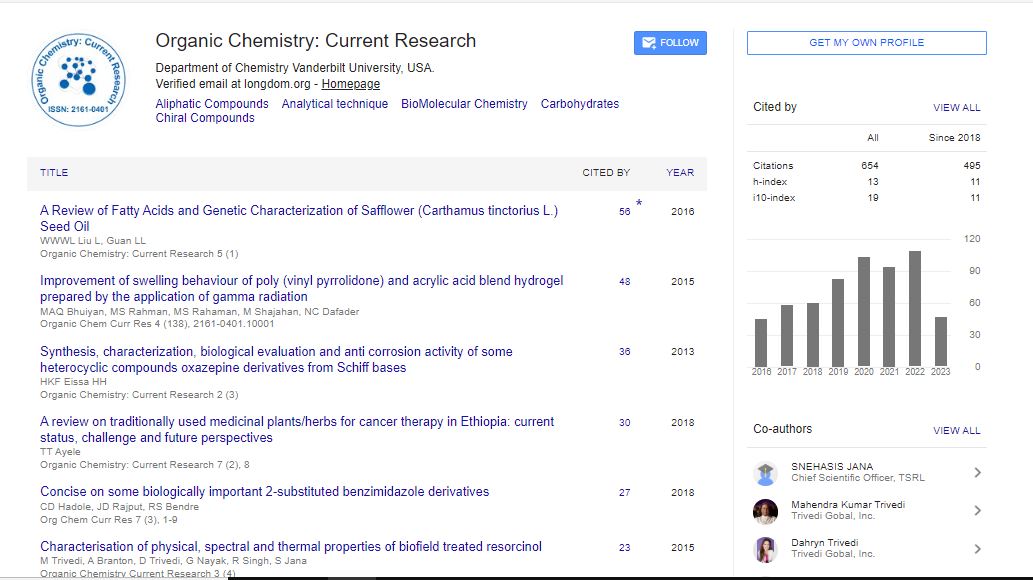This image features the home page for the Department of Chemistry at Vanderbilt University, USA, specifically highlighting the Organic Chemistry Current Research section. 

In the upper left-hand corner, there is a distinctive logo, a thin-lined blue circle set against a white background. Encircling the interior of this blue circle are the words "Organic Chemistry Current Research" in the same shade of blue, reminiscent of a family crest or various state and city seals. At the center of the circle is a smaller emblem, possibly representing a proton and neutron orbiting one another.

The page prominently displays a list of what appears to be research articles or titles of current research endeavors. Six different entries are visible, each associated with two additional categories: "Cited By" and the publication year. 

In the top right-hand corner, there is an option to "Get My Own Profile," inviting users to create their own profile. Below this, a graph displays data over different years, spanning from 2016 to 2023, with the year 2022 showing the highest values. 

The bottom right-hand corner of the page highlights co-authors, listing three individuals. Two of these co-authors have personal profile photos, while the third features a default image.